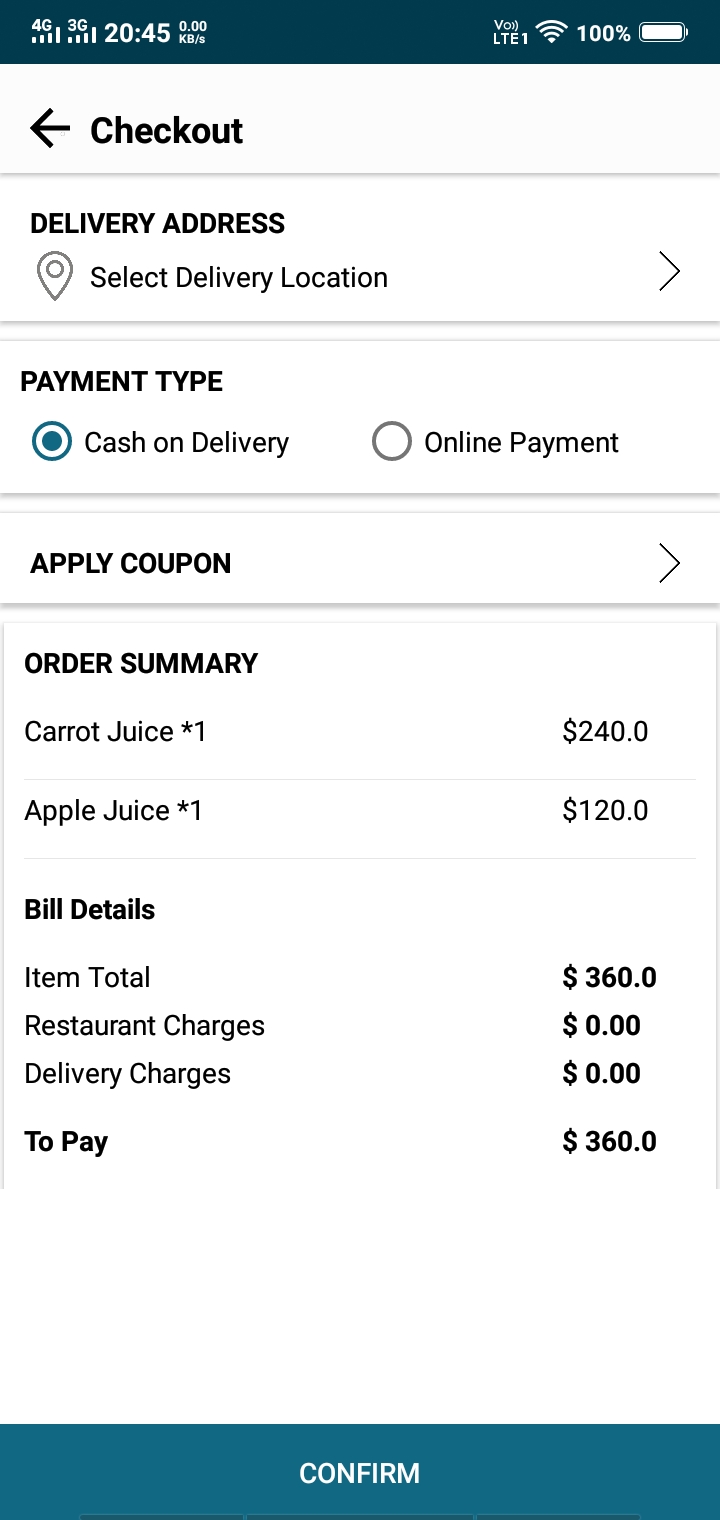The image displays a detailed screen from a mobile application, likely related to online food ordering. At the top, there are signal indicators including 4G, 3G, LTE, and Wi-Fi symbols, showing full connectivity. 

Beneath the signal icons, there are elements that describe navigation and transaction status, such as a left arrow indicating 'go back' and a 'checkout' option followed by a line heading. The section names 'Delivery Address' and 'Payment Type' appear next, suggesting user-selectable options. The payment options available include 'Cash on Delivery' and 'Online Payment,' with an icon next to each; the latter is likely highlighted or empty.

An 'Apply Coupon' button is present, paving the way to a detailed 'Order Summary' that lists the items ordered: Carrot Juice priced at $240 and Apple Juice priced at $120. Below the summary, 'Bill Details' break down the costs: the item total is $360, with no additional charges for the restaurant or delivery, making the total amount payable $360.

Finally, there is a prominent blue rectangle button labeled 'Confirm,' highlighted at the bottom of the screen. The overall layout suggests an intuitive user interface designed for a seamless ordering experience.